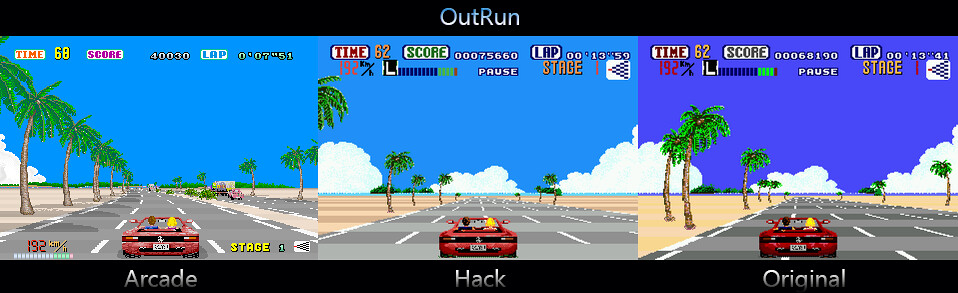The triptych illustration features a red cartoon car driving along a coastal road, surrounded by beach scenery on both sides. The car is occupied by two passengers: one with short blonde hair sporting a pink shirt and another with brown hair wearing a blue shirt. The road they travel on is depicted in a light gray shade with white demarcation lines and is characterized by shadows cast by palm trees lining both sides. In the first panel, an additional side street is visible, providing a more dynamic perspective that is absent in the subsequent panels.